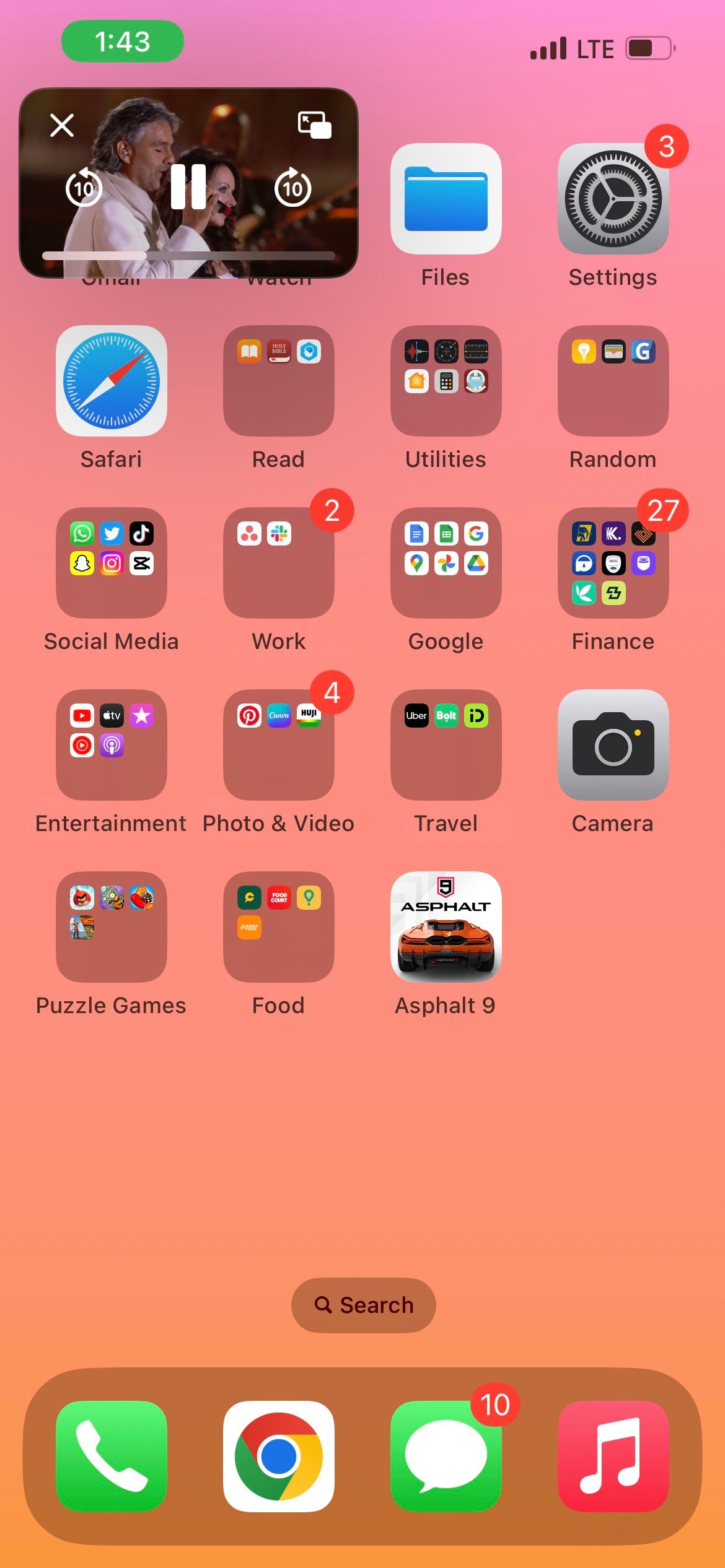This screenshot features a cell phone's home screen, showcasing its wallpaper and several organized folders. Prominently, a mini video player is positioned in the upper left corner of the screen. Within this player, two individuals are visible, both facing right. Predominantly, we see the right profiles of these figures, who appear to be performing on stage. The background of the video is blurred, hinting at another person playing a musical instrument. In the foreground, closest to the camera, is a male figure donning a white coat, holding a microphone in his right hand and seemingly singing. To his left and further back is a woman with black hair, visible in partial profile. The time, displayed at the top left of the screenshot, is 1:43, while the LTE signal indication is clearly marked in the upper right corner of the screen.